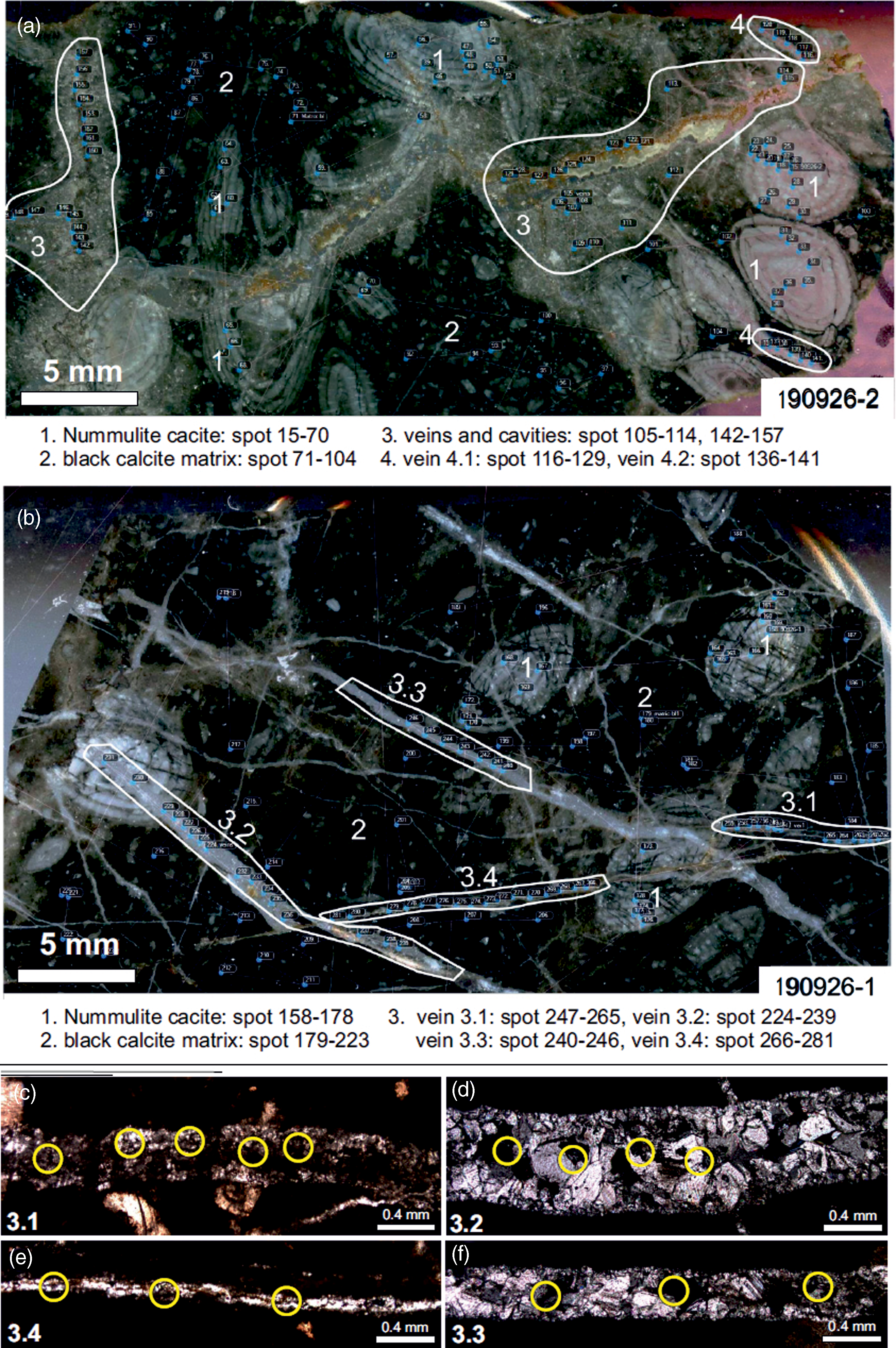This detailed image set appears to depict magnified views of geological samples, possibly minerals or rocks, and uses scales of five millimeters for reference. The primary image displays various features of the samples, enhanced with white outlines and labels for clarity. These features are numbered and identified as "Numulite Cassite Spot" for number one, "Black Calcite Matrix Spot" for number two, "Veins and Cavities" for number three, and "Vein" for number four. The image includes complex structures, some resembling pink blobby rocks, granite-like gray shapes, and darker inclusions, suggesting a detailed study of mineral formations. Below this main image, a secondary image with similar characteristics is mapped out and labeled, focusing on specific details within the sample. Further down, four smaller images highlight certain aspects with yellow circles, emphasizing particular spots within the larger images. The content, though intricate, aids professionals like geologists or medical imaging experts in analyzing the samples.